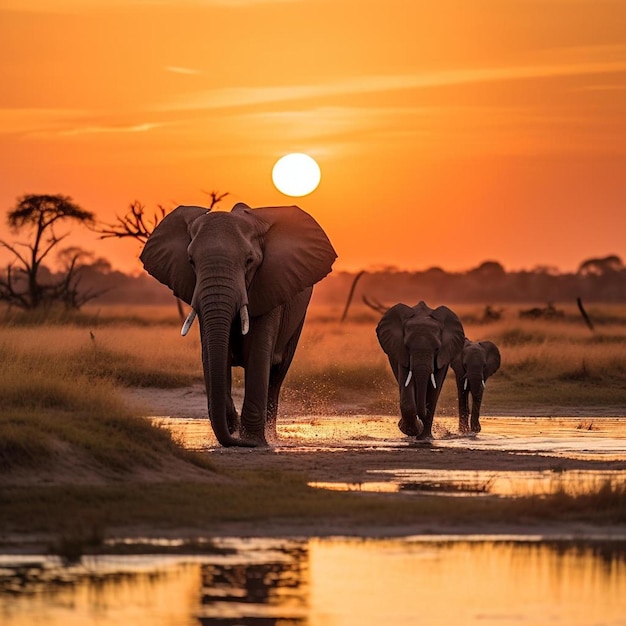In this mesmerizing outdoor scene set in Africa, three elephants—a large adult in the center, a slightly smaller juvenile to its right, and the smallest baby trailing behind—gracefully walk through shallow puddles, splashing water around their feet. The ivory tusks of the elephants are prominently visible against their gray skin. The setting sun, a bright ball of orange and yellow, casts a golden hue over the image, reflecting off the water and giving it a warm tint. The background features a blend of dark, sparse trees and tall grasses, framing the wildlife. A gentle incline with green grass leads up a small hill on the left, adding to the texture and depth of this safari scene. The vibrant orange sky enhances the beauty of this moment, capturing the essence of wildlife photography.